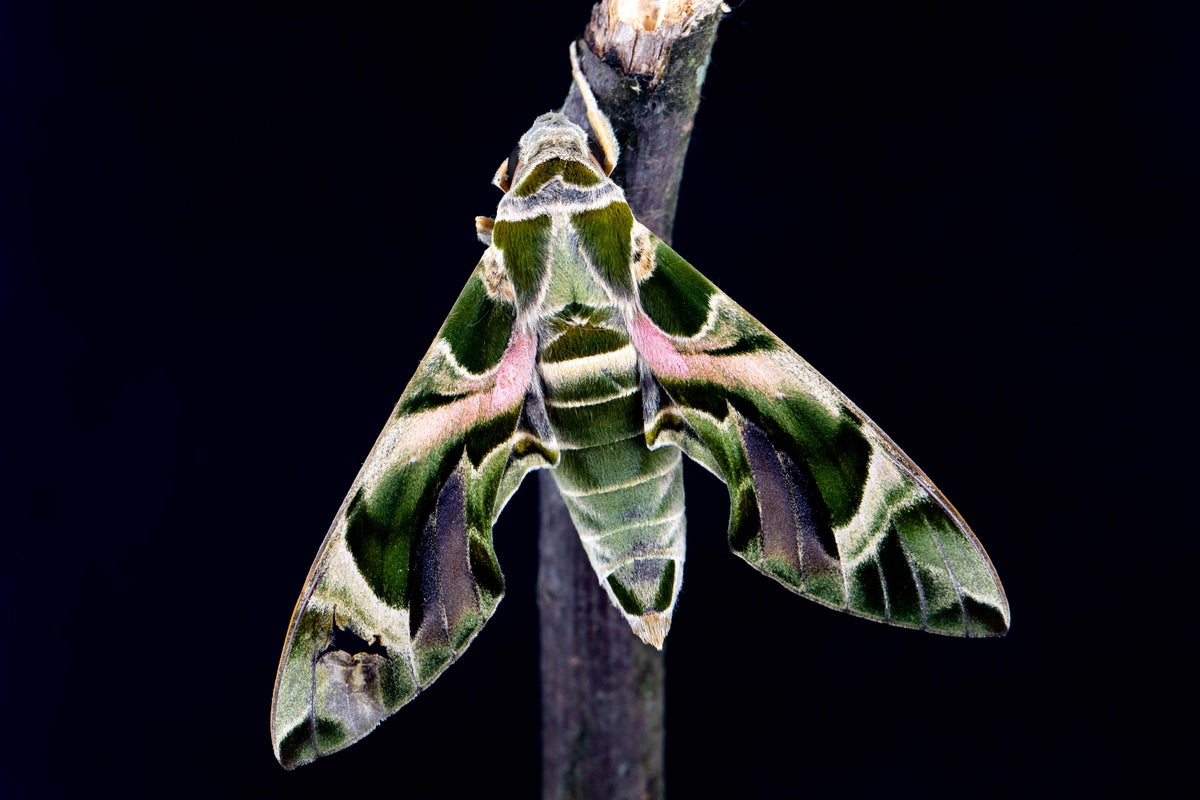This image is a high-contrast, close-up photograph of a moth, possibly a luna moth, set against a jet-black background. The intricate and vivid details of the moth are accentuated, likely through digital alteration to enhance contrast and saturation. Facing upwards and slightly tilted to the left, the moth showcases its mottled wings and back, displaying a striking array of colors, including dark green, black, white, pink, and purple. A delicate pattern of stripes extends beyond its wings onto its body, where the fine hairs on the back of its head are visible. The moth rests with one leg outstretched on a twig that runs centrally through the image. The twig, which displays a noticeable break at the top center, curves slightly and is rendered in a nearly black, purplish hue. The image offers a detailed and vibrant study of the moth’s unique patterns and textures, set against the stark simplicity of the dark background.